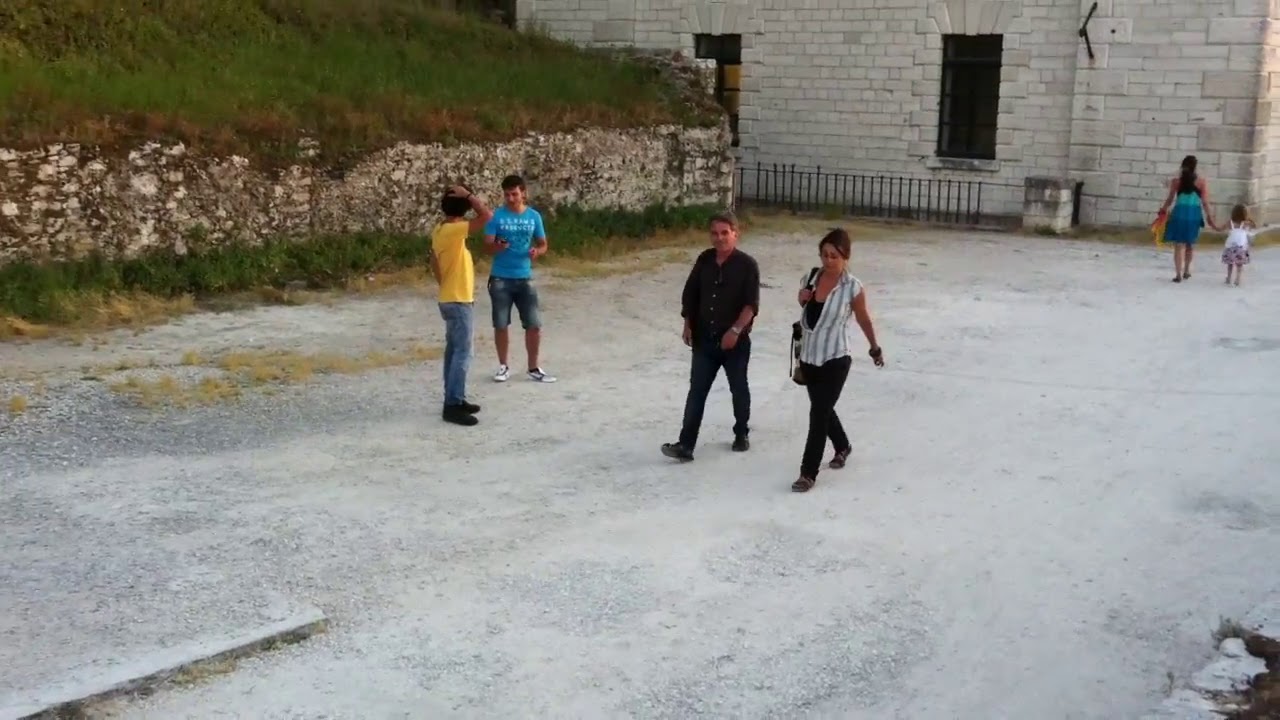The outdoor image depicts a bustling scene on a gravel and dirt pathway. Central to the photo is a couple walking together. The woman is in a white blouse with gray stripes over a black tank top, paired with black pants. She carries a handbag over her shoulder and looks down as she moves forward. Beside her, on her right but our left, is a man dressed entirely in black—black shirt, black pants, and black shoes; he has slightly grey hair, rolled-up sleeves, and is wearing a wristwatch, stepping with one foot forward.

To their left stand two young men engaged in conversation. One, nearer to the couple, wears a blue shirt with white text, blue jean shorts, and sneakers. His companion, closer to the left edge, sports a yellow t-shirt, blue jeans, and black shoes, with one hand resting on the back of his head.

In the top right corner of the scene, a woman in a blue gradient dress walks away, holding the hand of a little girl who wears a white dress. They head towards a light stone building in the background. Adjacent to this building is a stone wall topped with grass and various shrubs growing at its base. The entire backdrop sets a quaint, slightly Middle Eastern ambiance to this active walkway scene.